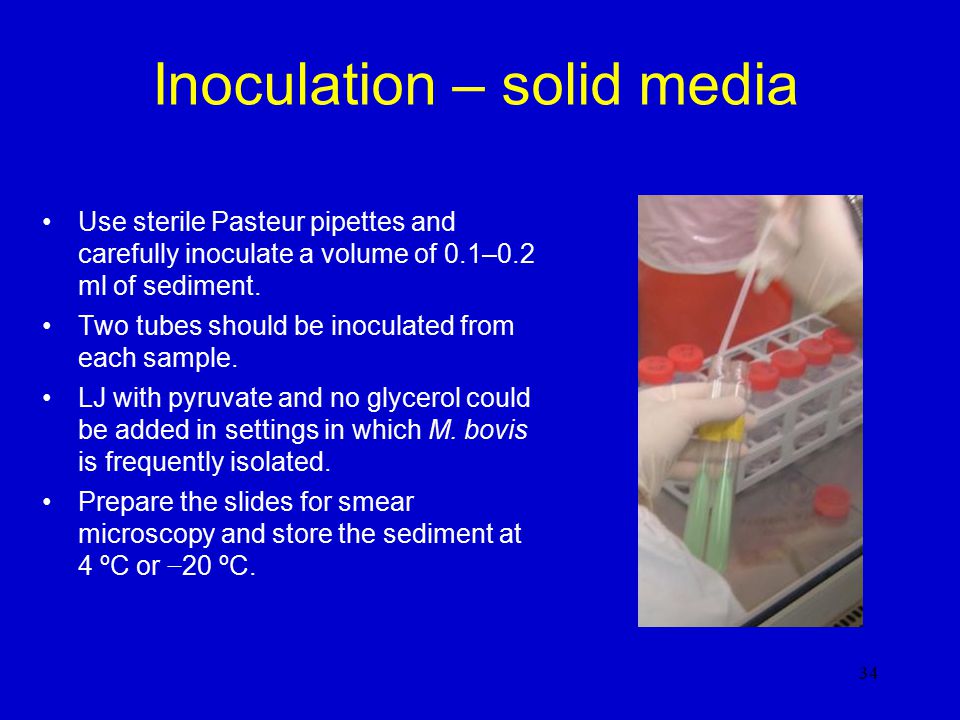The image appears to be from a PowerPoint presentation or instructional manual focused on biology lab procedures. The background is solid bright blue, with a yellow title at the top reading "Inoculation - Solid Media." Below the title, white text details the steps for a specific inoculation procedure. The instructions include four bullet points: (1) Use sterile pasteur pipettes and carefully inoculate a volume of 0.1-0.2 ml of sediment. (2) Two tubes should be inoculated from each sample. (3) LJ with pyruvate and no glycerol could be added in settings where M. bovis is frequently isolated. (4) Prepare slides for smear microscopy and store the sediment at either 4 degrees Celsius or -20 degrees Celsius. On the right side of the slide, there's an image of a pair of gloved hands holding two test tubes while using a pipette with a white tip to inject a substance, which appears to be green liquid, into one of the test tubes. This comprehensive visual and textual guide provides a clear overview of the inoculation process in a laboratory setting.